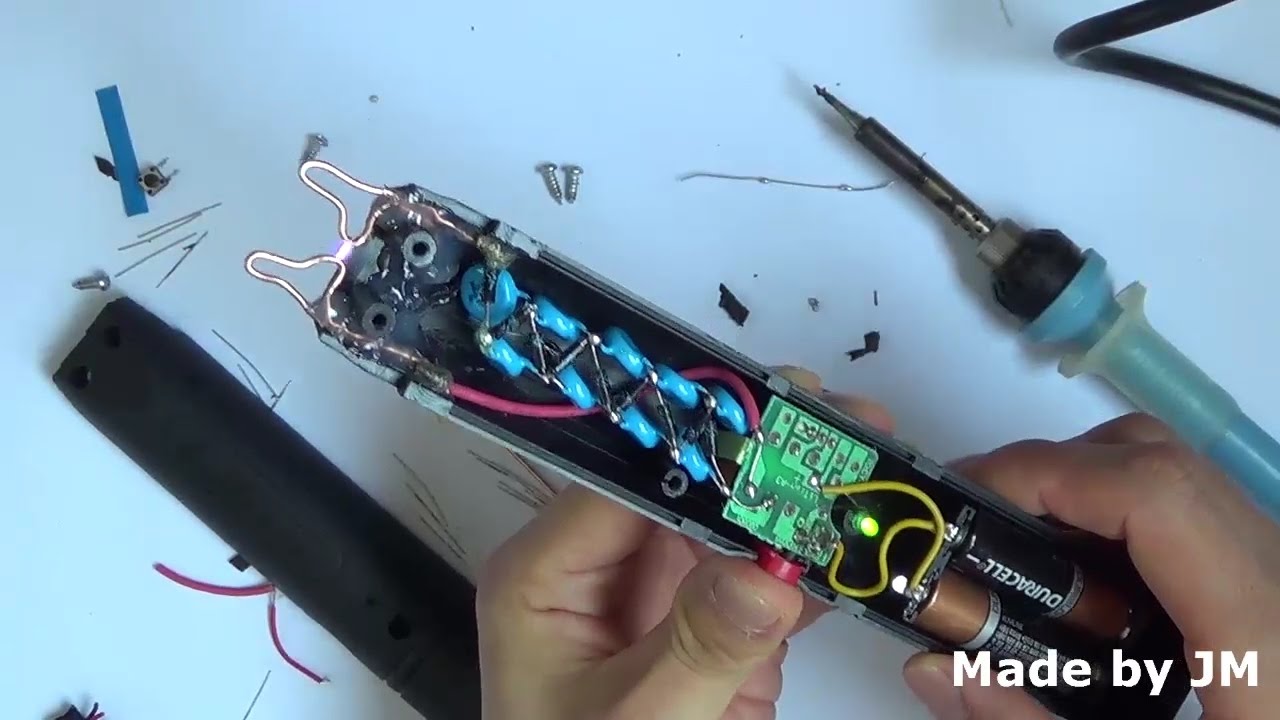The image features a pair of hands holding a disassembled electronic device, resembling a remote control. The remote's internals are exposed, revealing a green chipboard centrally positioned, complemented by blue capacitors at the top and a couple of Duracell batteries. To the right of the hands, a soldering iron with a bluish handle and a black cord is visible, suggesting an ongoing repair. Scattered around the scene are several screws and the remote's dark gray or black back cover. Additionally, red wires extend from the device, connecting various components. The setup rests on a blue-white table, with the phrase "made by JM" in white font on the far right.